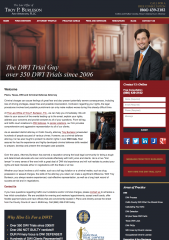This screenshot captures the homepage of a legal or lawyer's website. At the very top, a black navigation bar spans the width of the screen, exhibiting the law firm's or lawyer's office name in white text on the left, though the text is somewhat blurry. On the right side of this bar, a contact phone number is displayed, also in white. Directly beneath this, a red navigation bar contains eight white-link buttons, though the specific labels are indistinct.

Below the navigation bar, a prominent banner extends across the screen, featuring a lawyer or possibly the website's spokesperson. He is depicted in a black suit paired with an orange tie, positioned on the right side of the banner. The background appears to be the interior of a courthouse, complete with wooden paneling, the judge's bench, and an American flag, enhancing the legal ambiance.

To the right of the banner, there is a red column containing a white contact form, inviting visitors to reach out for more information or services.